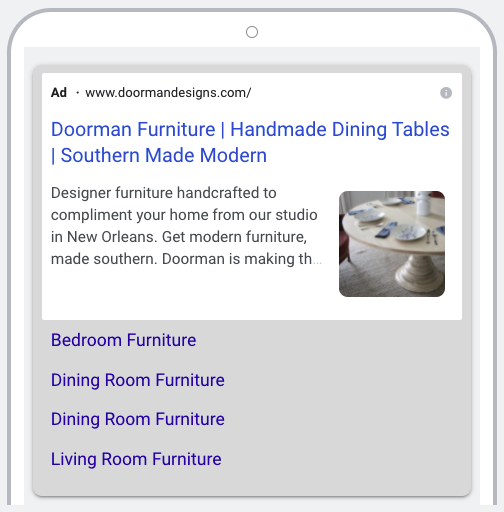This image is a screenshot from a mobile device, showcasing a search result for furniture. The search query includes categories such as bedroom furniture, dining room furniture, and living room furniture. Featured prominently in the screenshot is an advertisement from www.doormandesigns.com, specifically for Doorman Furniture. The ad's text highlights "Handmade Dining Tables" and describes the furniture as "Southern Made Modern," emphasizing that the designer pieces are handcrafted to complement homes, crafted in a studio located in New Orleans. The tagline "Get modern furniture made southern" is partially visible, cutting off with "Doorman is making the..."

Accompanying the text is a small image of a dining room table. The table is off-white with a pedestal base, elegantly set with plates, napkins, and silverware, capturing the essence of the advertised handcrafted aesthetic.